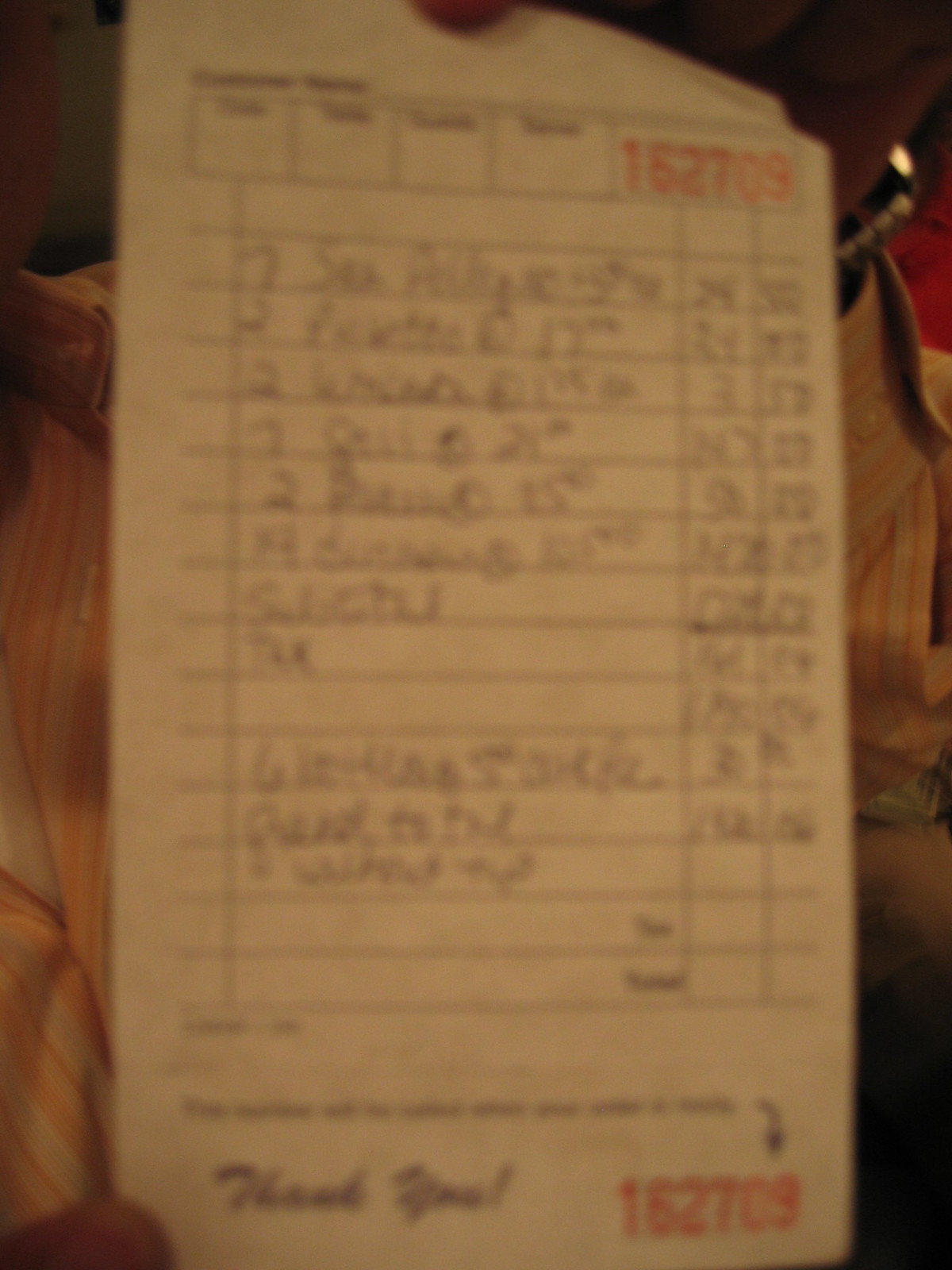A vintage, itemized receipt held by a person is the focal point of this photograph. The image is noticeably blurry, making the handwritten details on the receipt largely indecipherable. Despite the blur, the receipt features prominently printed red numbers "162709" at both the top and bottom right corners. The person's hand is visible holding the receipt, and in the background, there is a glimpse of their striped shirt, collar, and the lower part of their face. The receipt showcases several rows and columns with handwritten entries listing items, individual prices, and total amounts. At the bottom of the receipt, "Thank you" appears in an elegant cursive font.